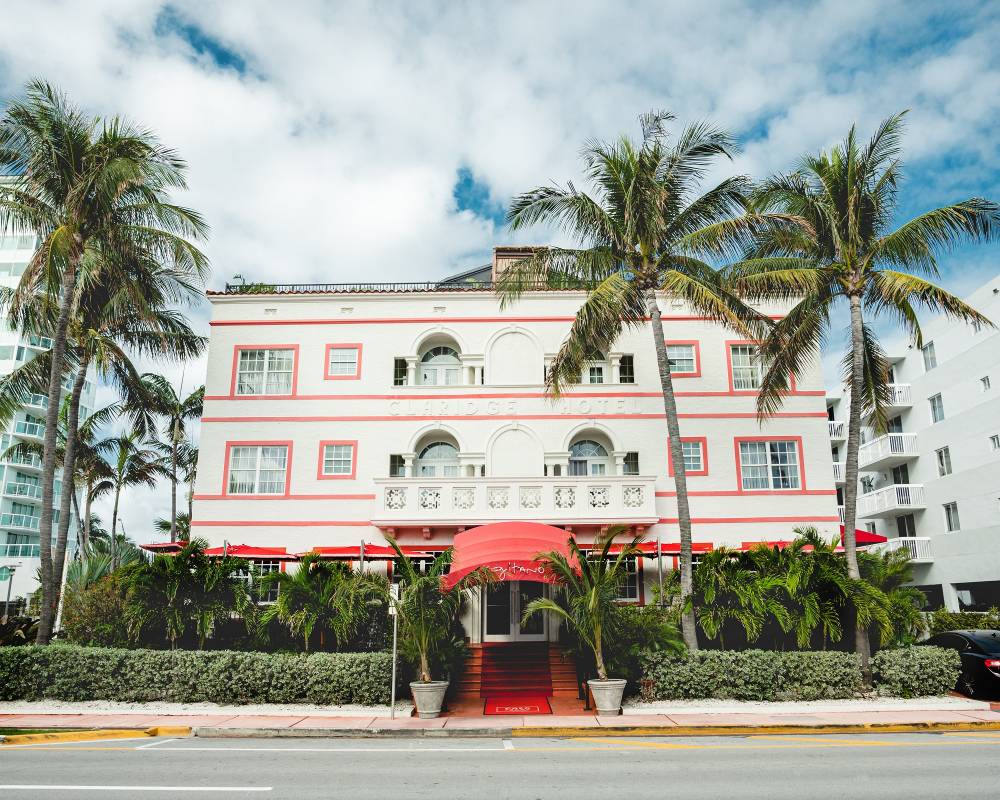The image shows the exterior of a white three-story hotel or restaurant, adorned with red trimming around the windows and the top of each floor. A red awning and a red carpet lead to the entrance, which is flanked by two large potted plants. The scene, set during the daytime, features a partly cloudy sky with patches of blue. On the left side of the building, there are two large palm trees and three smaller ones, while on the right side, two more tall palm trees can be seen. Various trees and neatly trimmed bushes surround the building, contributing to its lush appearance. To the left of the main building stands a tall white high-rise, and on the right, a shorter white building, possibly an apartment complex. The overall setting suggests a warm, tropical location, likely Miami or California.